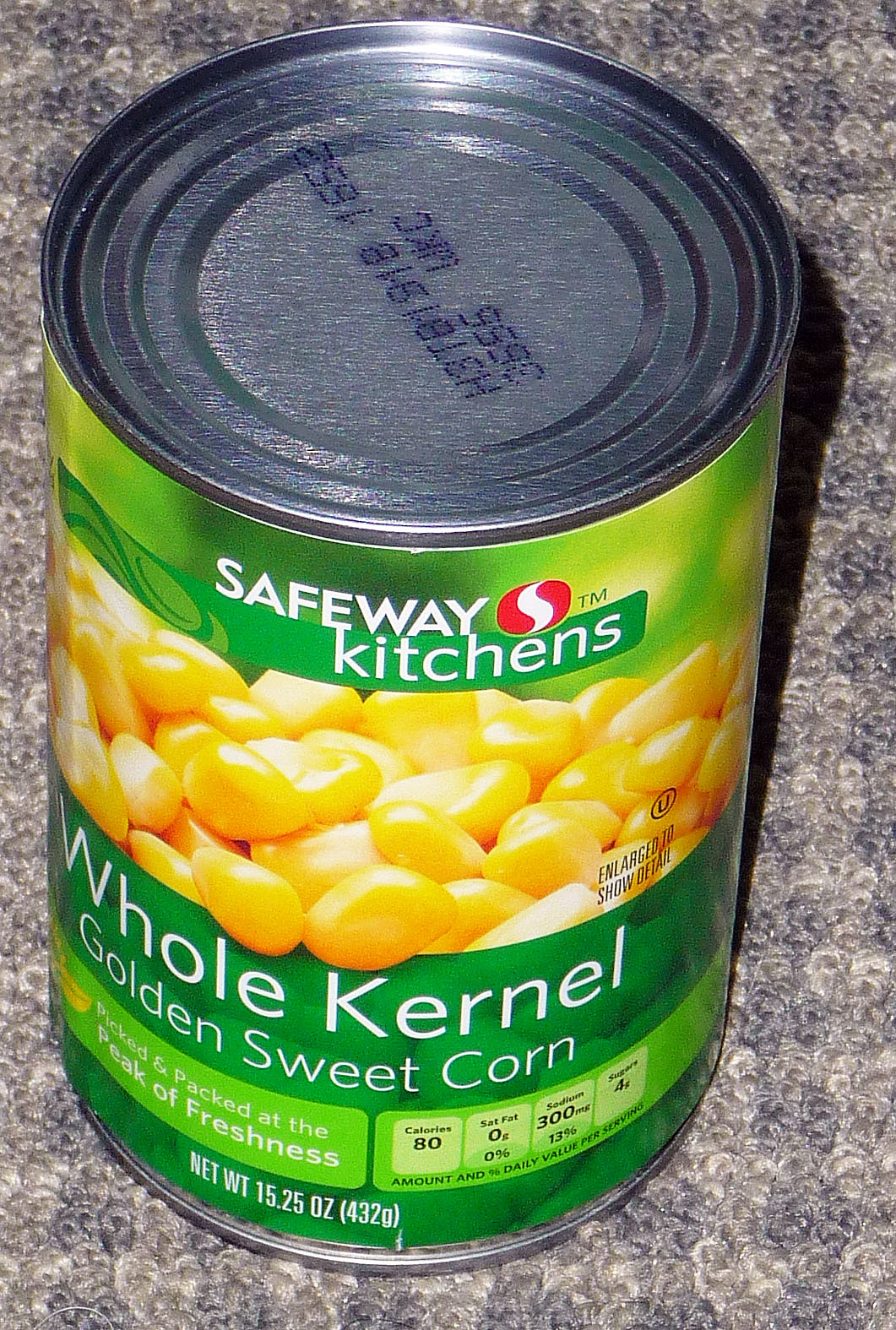This vertically-oriented color photograph offers a close-up view of a can of whole kernel golden sweet corn, prominently marked with a "Safeway Kitchens" label at the top. The can sports a bright green label featuring an appetizing image of vibrant yellow corn kernels in the center, surrounded by additional text that sits on a lighter green banner proclaiming, "Picked and packed at the peak of freshness." The bottom of the label displays, in white letters against a black-green background, the product name: "Whole Kernel Golden Sweet Corn." On the right side of the can, a dedicated panel provides nutritional details including daily values and caloric information. The top of the can, positioned slightly angled from above, reveals a faintly printed date and batch stamp in dark blue text. The entire can rests atop a light blue and white rug with a delicate, plaid-like pattern, providing a cozy backdrop to the image. The net weight of the product is clearly indicated at the very bottom of the label, stating 15.25 ounces.